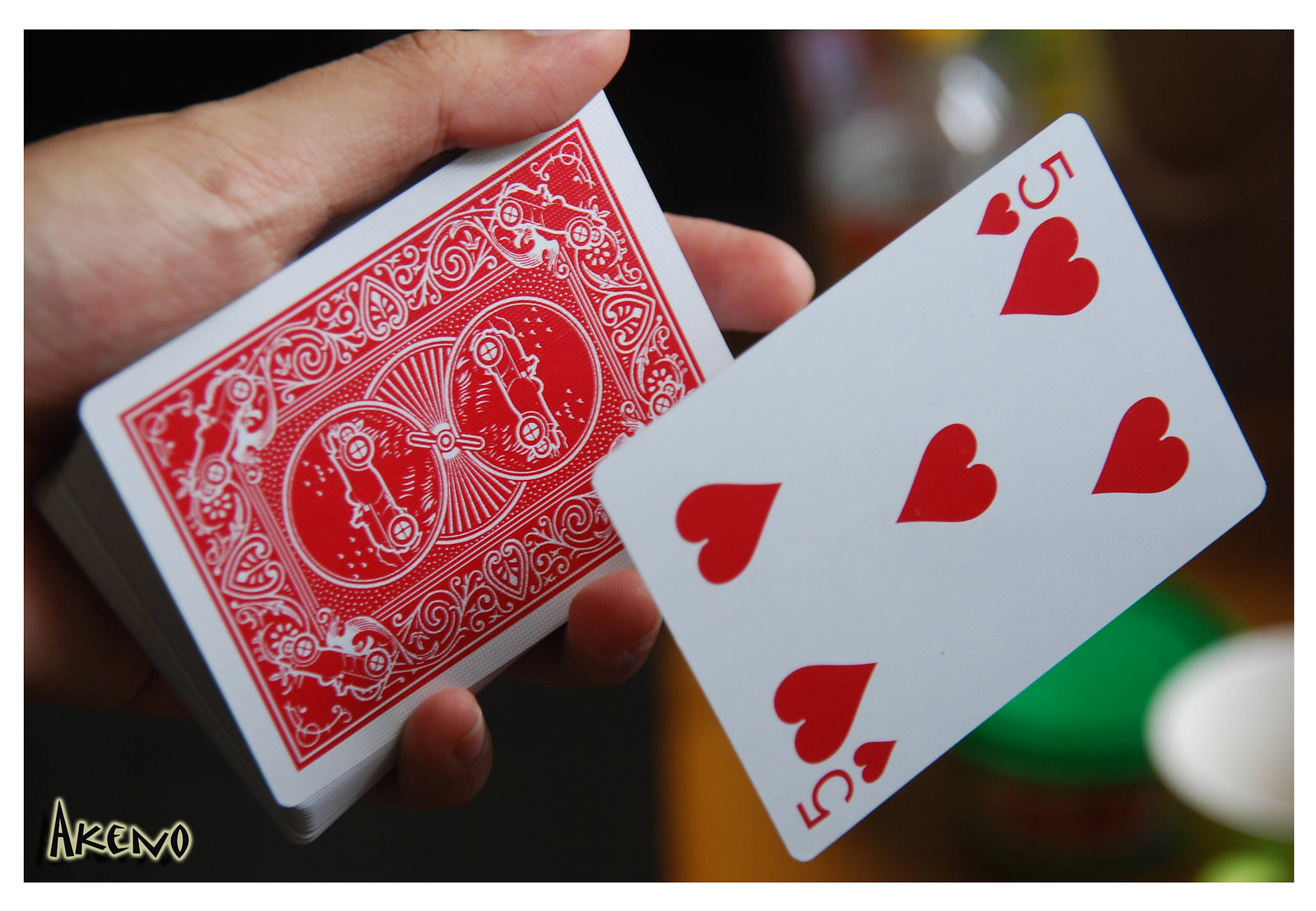Here's a cleaned-up and detailed caption for the described image:

---

In the image, a hand is holding a deck of red-backed playing cards, arranged face down. The detailed scrollwork on the back of the cards features intricate designs, including small heart motifs and two circular areas resembling speedometers with car images facing different directions. This decorative style is reminiscent of traditional Bicycle cards, although the exact brand is not identifiable from this view.

The focus of the image is on the five of hearts card, which appears to be levitating above the deck, creating the impression of a magic trick. This card is slightly to the right of the screen and is face-up, showcasing its red heart symbols.

The background is heavily blurred, offering only vague hints of colors and shapes, including white, green, and a wood-like hue, making it difficult to discern the location. However, the lettering "A-K-E-N-O" is clearly visible in the bottom left corner, written in black letters with yellow outlines.

Overall, the sharp contrast between the clear depiction of the cards and the indistinct background creates an intriguing visual effect, emphasizing the floating card and the mysterious ambiance of the scene.